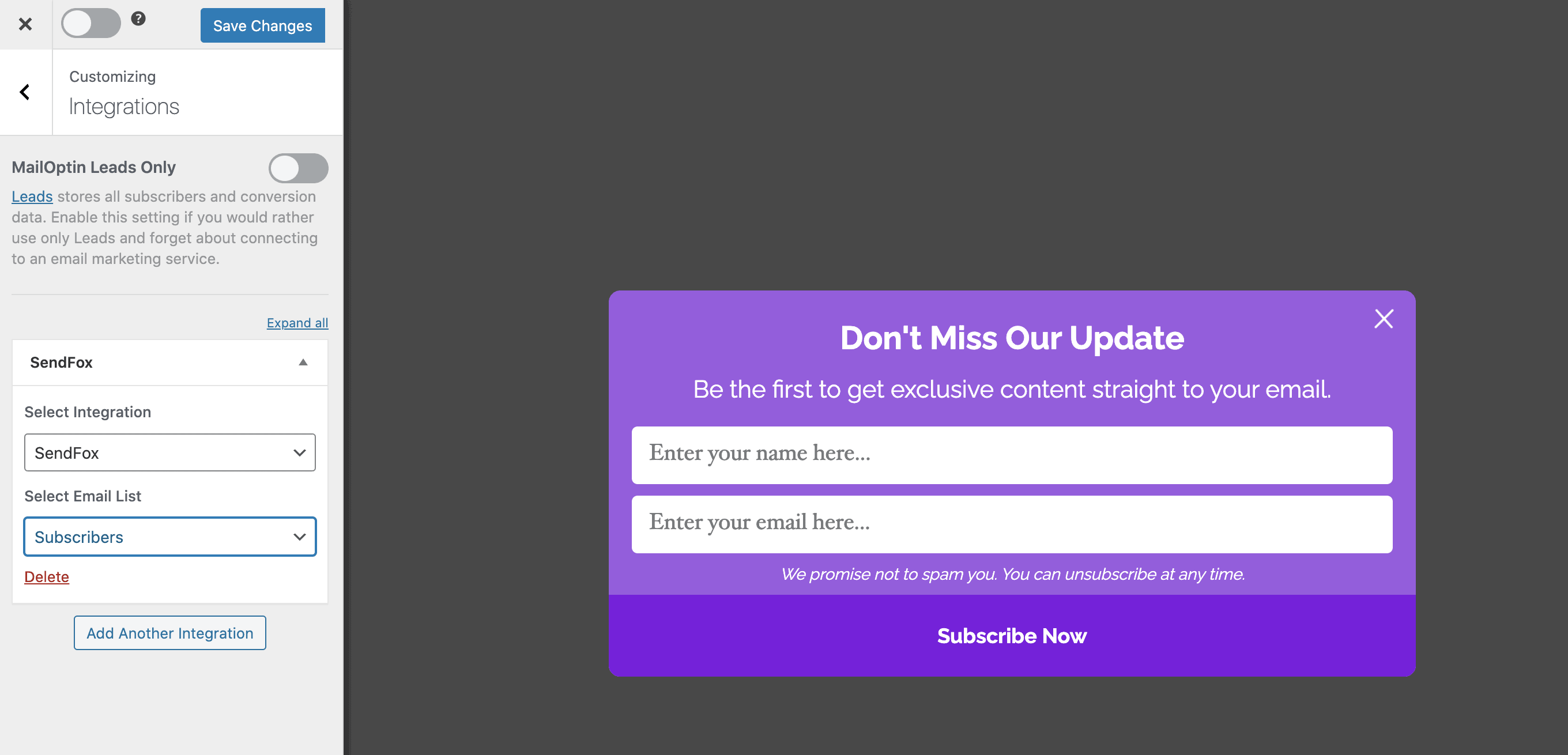The image features a centered pop-up screen against a black background with a prominent message in white text: "Don't miss our update." Directly below, another line of text reads, "Be the first to get exclusive content straight to your email." The pop-up includes two white rectangular input fields; the first is labeled "Enter your name here" and the second below it, "Enter your email here." At the bottom of the pop-up is a darker shade of purple button with "Subscribe Now" written in white.

On the left side of the image, there is a vertical panel with a grey base color and white sections containing various controls and information. Starting from the top left corner, there is an X button followed by a toggle button. To the right of these buttons is a blue "Save changes" button. Below these controls, a section is labeled "Customizing Integrations." Underneath is an "Mail opt-in leads only" toggle, which is switched off, accompanied by some small text with additional information. Further down, there are labels such as "BendFox" and "SandFox," with a drop-down menu below labeled "Select Email List," currently set to "Subscribers."

At the bottom of this panel, there is a red "Delete" button followed by a light blue "Add Another Integration" button. The left panel contrasts the grey background with white sections to neatly segment the various control and information areas.